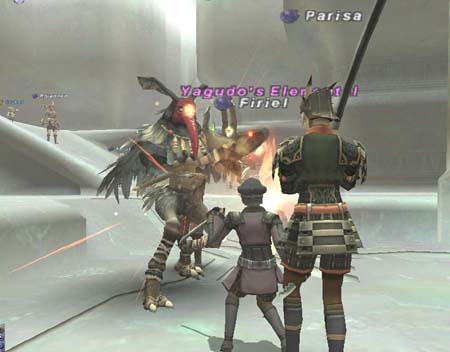This video game screen capture features a detailed and dynamic scene. In the foreground, two figures stand with their backs to us, facing a monstrous creature. The shorter figure, located in the center lower half of the image, is clad in purple armor and holds a thin blade, with their left arm bent at the elbow. Closer to the right and occupying more of the foreground is a taller, adult-sized figure dressed in green armor. This character wields a large sword that extends from their upper torso and exits the image towards the upper right.

Slightly left of center and further back, a monstrous humanoid bird-like creature stands menacingly. The creature possesses clawed feet, long ears, a trunk-like appendage resembling an elephant's, and a bright orange beak. The scene suggests a battle scenario, as the armored figures appear to be engaged with this monster, which might be labeled "Yagudo's Elemental Firiel" per the obscured in-game text.

The environment around the characters is silvery and structured, featuring large, windowless white walls. There is a ramp descending from the left, upon which another figure is visible. Above this dynamic scene, white and purple text reads “Parisa” and “Yagudo’s,” respectively, hinting that this could be an online or collaborative fantasy video game. The overall setting includes several platforms interconnected by ramps, contributing to the strategic layout of the battlefield.